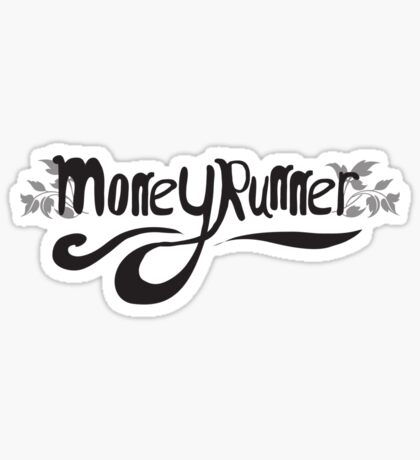This graphic illustration features the text "Money Runner" prominently in the center, rendered in black, extravagant, and stylized script on a light gray background. The "M" and the final "R" each have gray plant illustrations sprouting from their edges. The "Y" in "Money" is particularly large and loops upward to seamlessly form the "R" in "Runner." Both words are underlined: "M-O-N-E" has a subtle underline while "Runner" has a matching one. The entire logo, resembling a sticker, is outlined with a delicate gray line, adding cohesion to the composition.